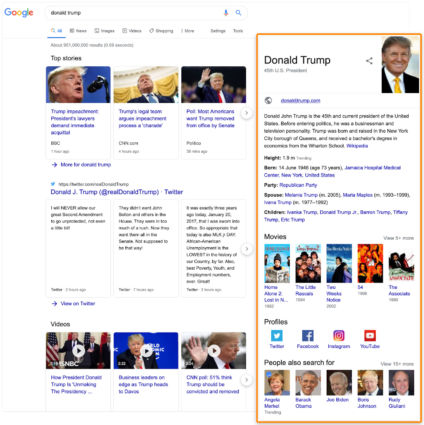This image showcases a Google News page prominently featuring Donald Trump. Detailed content includes a variety of articles related to Trump, accompanied by a list of five popular movies. The page also highlights related search topics under "People also searched for," and displays icons for major social media platforms such as Twitter, Facebook, Instagram, and YouTube. Notably, it features Donald Trump's active Twitter feed. The page offers playable video clips and includes a summarized Wikipedia entry on Trump. Additionally, there is a section displaying an image of Barack Obama, providing a well-rounded view of the type of content and navigation options typically available on Google News when focusing on a notable public figure.